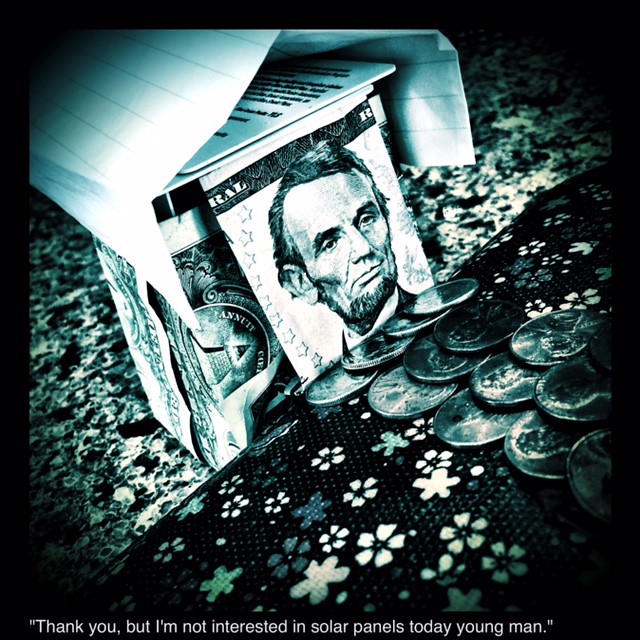The image depicts an intricate piece of artwork featuring a house constructed out of American cash. The front of the house displays a folded five-dollar bill showcasing Abraham Lincoln's face, and the sides and back are formed using one-dollar bills. Resting on top of the structure is a folded piece of white binder paper, creating an A-frame roof, with two credit cards laid flat on it. Quarters are arranged in rows of three or four, possibly resembling a walkway, and the entire setup is set against a fabric backdrop decorated with flowers. The colors in the image primarily consist of black, white, shades of gray, green, and silver, with some faded hues as well. At the bottom of the image, the text reads, "Thank you, but I'm not interested in solar panels today, young man." The artwork, roughly five by five inches in size, appears to be crafted for an artistic message likely intended for social media sharing.